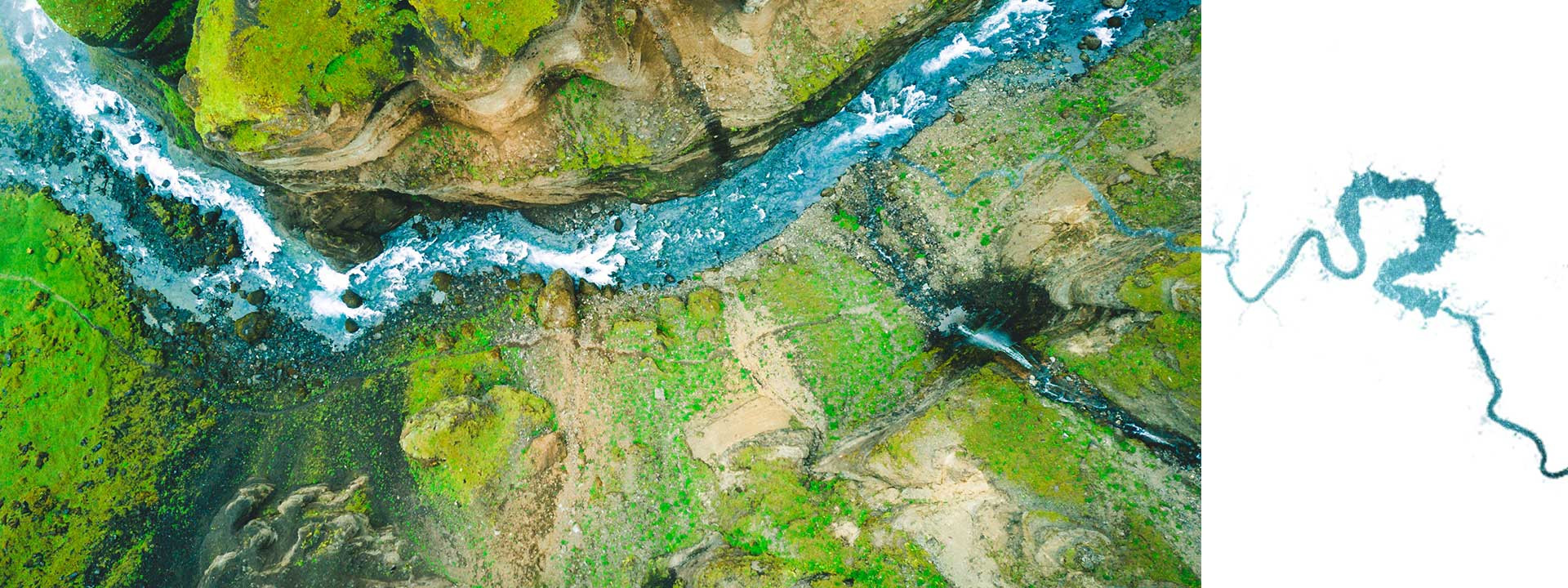The image is an overhead, aerial photograph capturing a vividly colored river meandering through a mountainous landscape. The river, a strikingly vibrant blue, starts from two points that merge into one before branching off again into a larger stream and two smaller ones. One of the smaller streams extends past the edge of the photograph, curving upwards in a horseshoe shape onto a white background in a unique artistic flourish. Encircling the river are cliffs adorned with bright, almost lime-green grass, interspersed with patches of brown, possibly indicating areas of drought. The land features rocks and dirt paths, adding texture to the scenery. On the right side of the river, a waterfall cascades down a high mountain range, leading to white foamy areas in the river, suggesting a fast current flowing over rocks. The riverbank includes a small gravel island with a few trees, surrounded by pale soil and greenery, creating a picturesque, dynamic landscape. The setting, possibly in spring, under a warm, daylight sky, gives the overall impression of a vivid, lively scene frozen in time.